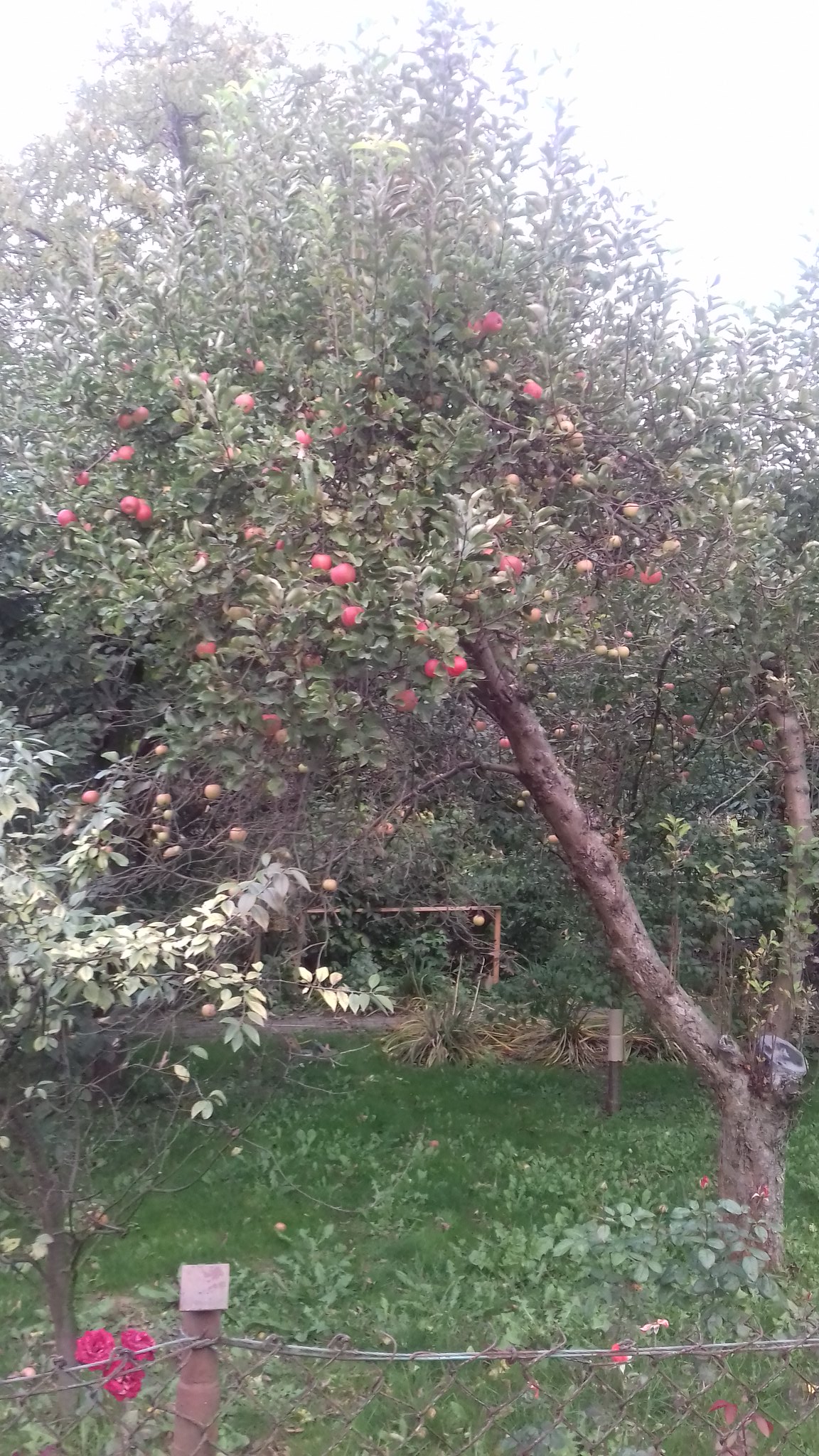This vertically-oriented photograph captures a lush, green outdoor scene, likely a backyard or garden. Dominating the image is a large apple tree, characterized by its brown trunk and branches laden with bright red apples. The tree leans noticeably to the left, extending from the bottom right towards the top left of the frame. The background features additional trees and shrubs, adding depth to the verdant landscape. The grass below the trees is somewhat overgrown, dotted with a mix of small plants and bushes. 

In the foreground, a wooden post marks the beginning of a wire fence, adorned with a few red flowers resembling roses. Near this post, a small sign is visible, though its text is indiscernible. Elements of the photo hint at a well-aged and somewhat unkempt garden setup, including what seems to be an old swing set or trellis in the distance. The vibrant colors of the green foliage and red apples, contrasted with the earthy tones of the tree trunk and branches, enrich the overall lively and dynamic composition of the scene.